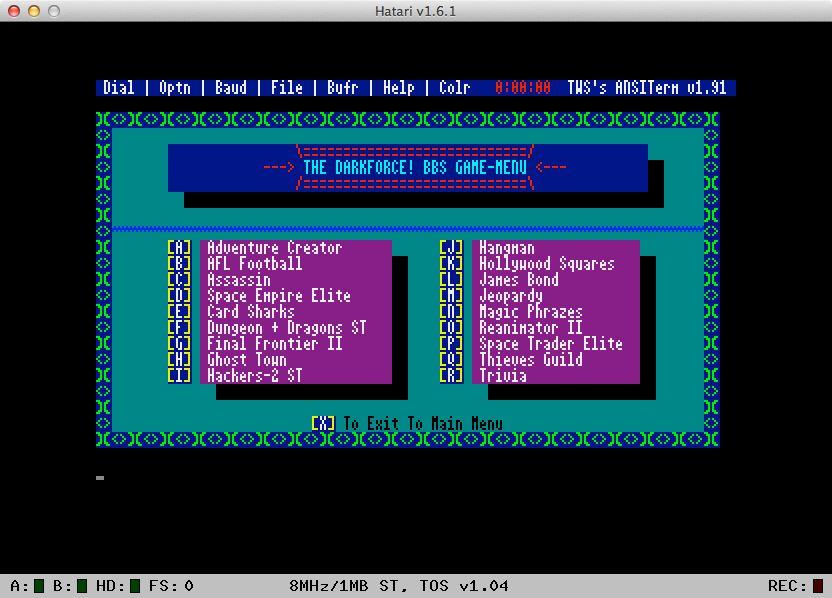The image depicts a computer desktop screen featuring a BBS (Bulletin Board System) game menu from a gameplay session. The entire background of the screen is solid black, but a large blue rectangle with a patterned border dominates the majority of the screen. At the top of this blue screen are the words "The Dark Force BBS Game Menu" in all caps, written in a teal-colored font. Below this, the interface showcases two purple square sections. The first purple square lists the letters A through I along the left-hand side and contains white writing for game titles like "Adventure Creator," "AFL Football," "Assassin," "Hangman," and "Hollywood Squares." The second purple square displays the letters J through R on the left side and includes games such as "Space Empire Elite," "Card Sharks," "Dungeons and Dragons," "Final Frontier 2," "Ghost Town," and "Hackers 2." Both purple squares are filled with a variety of additional game names in white font. At the very bottom of the blue screen, there is an "X" with the instruction "To exit to main menu." The top of the computer desktop screen shows a standard menu bar with the red X button, the yellow minimize button, and a clear button for managing the window.